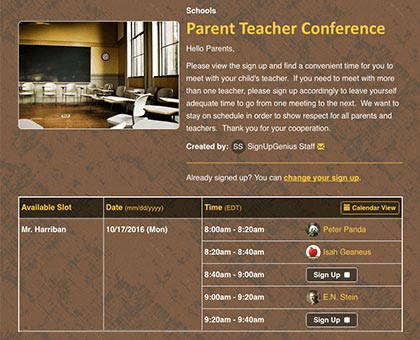This screenshot showcases a digital sign-up sheet for a Parent-Teacher Conference against a dark brown, textured background. The top-left corner features a photograph of a classroom filled with multiple desks and chairs, and a blackboard gracing the back wall, capturing a traditional educational environment. 

The text at the top reads, "Schools, Parent Teacher Conference. Hello parents. Please be able to sign up and find a convenient time for you to meet with your child's teacher. If you need to meet with more than one teacher, please sign up accordingly to leave yourself adequate time to go from one meeting to the next. We want to stay on schedule in order to show respect for all parents and teachers. Thank you for your cooperation. Created by Sign Up Genius staff."

The sign-up slots detail the available times for meetings. The list includes:
- Mr. Harabin on 10-17-2016 (Monday) from 8:00 AM to 8:20 AM EDT.
- Peter Perita from 8:20 AM to 8:30 AM.
- Isa Jodeas from 8:40 AM to 9:00 AM.
- E. N. Stein from 9:20 AM to 9:40 AM.

An additional note specifies the absence of plants, flowers, trees, and automobiles in the image. Touches like "Available slot" and "Sign Up" options underline the functional aspect of this digital tool, facilitating parent-teacher scheduling.